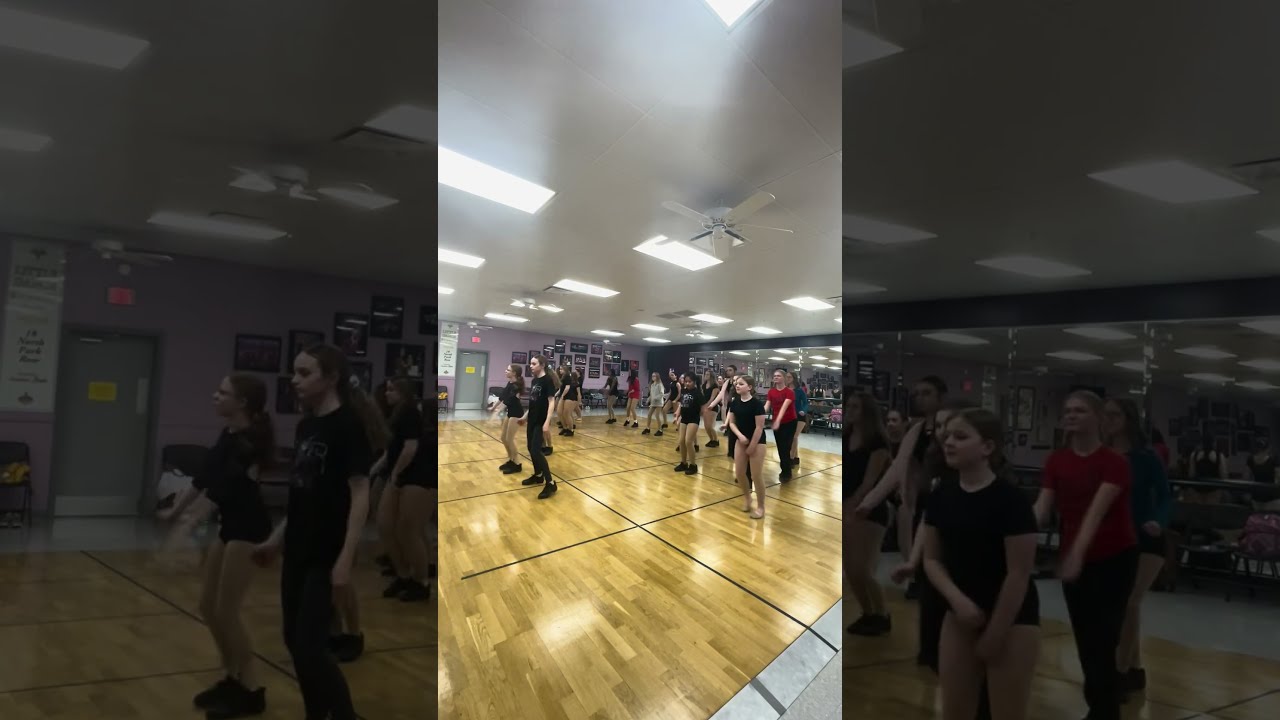The photograph captures an indoor dance studio divided into three vertical sections. The central image, framed by two enlarged and darkened versions on either side, showcases a brightly lit space with fluorescent lighting and ceiling fans. The studio features a shiny, hardwood floor marked with black grid lines creating large boxes. The back wall of the room is lined with large mirrors, while the left-hand wall is painted purple and adorned with numerous photos.

The dance studio is occupied by a group of about a dozen young women and girls, most of whom are positioned with knees slightly bent and one foot raised, seemingly engaged in dance practice. They are dressed in various gym and dance outfits, predominantly black dance shoes. The attire ranges from black leotards and skin-toned tights paired with black tops and shorts to sweatpants and sweatshirts. Notably, one girl in the center stands out wearing black pants and a pink hoodie. The group appears to be focused and coordinated, each facing slightly to the side, contributing to the dynamic atmosphere of the dance session.